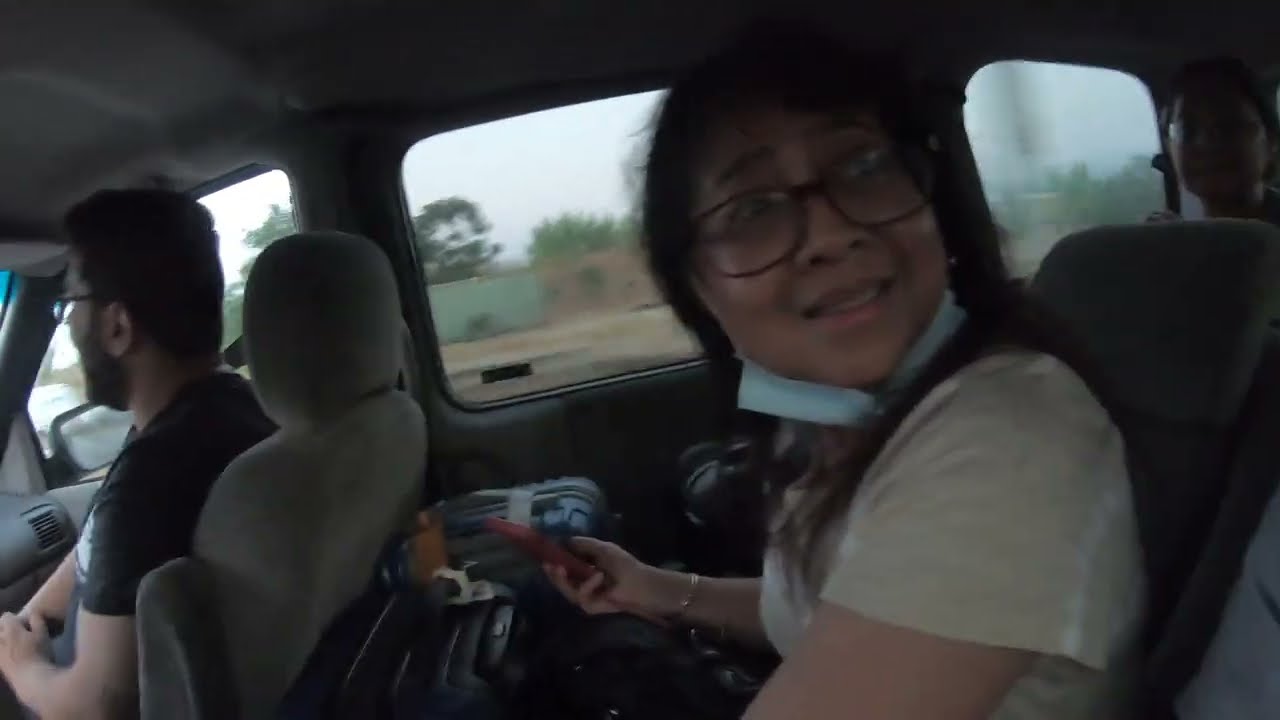The photo, taken from the backseat interior of a car, captures a detailed scene involving two passengers. Closest to the camera, a woman is seated in the backseat, making a grimace. She has long hair and is wearing red-rimmed glasses. Her blue cloth mask is pulled down under her chin, revealing her slightly open mouth that conveys a worried expression. She is dressed in a tan-colored t-shirt with white stripes and sports a bracelet on her right hand, which also holds a red carrot-shaped object, possibly a phone with a red cover.

To her right, there are two pieces of luggage – one blue and the other black. Seated in the front right passenger seat is a man with a beard and mustache. He is wearing black sunglasses and a black t-shirt, secured by a seatbelt. The vehicle has cream-colored seats and possibly a third row, though it is only faintly visible. Through the windows, we catch glimpses of the outside environment, including small houses, trees, and the sky.